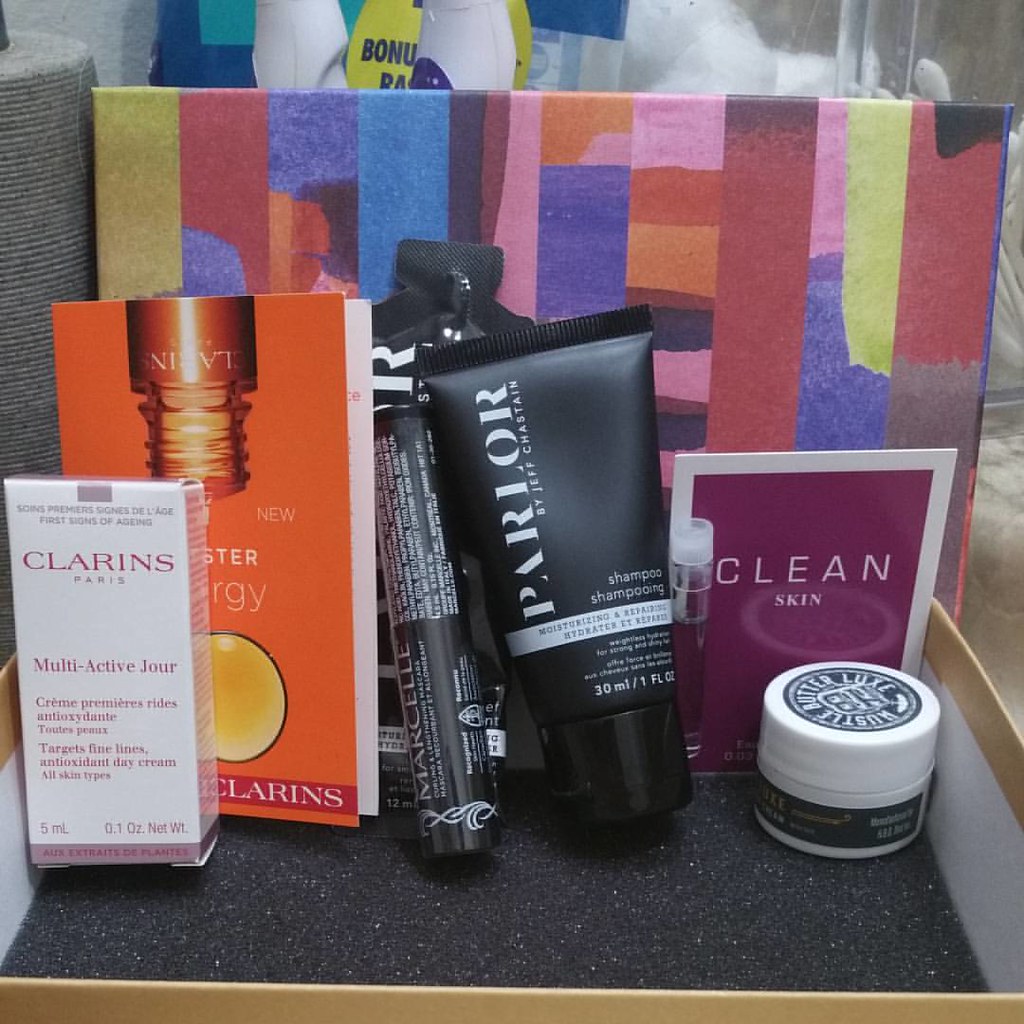In the image, a collection of beauty products, creams, and lotions are carefully arranged within a tan ridged box with a white interior. The box's lid, which is now placed upside down, features a gray foam pad housing several of these beauty items. Behind the displayed products stands a vertically positioned, multicolored abstract artwork that appears to be the cover of the box.

From left to right, the products include a smaller rectangular white box with white lettering, titled "Clarins Paris Multi-Active Jour," detailing its features. Next to it, there is an orange pamphlet featuring an image of an upside-down container spilling some lotion. Following that, there's a black tube with white writing and a black gel dispenser. The arrangement concludes with a small white tub, adorned with dark green stickers. The composition of the image highlights the diverse array of beauty offerings in an aesthetically pleasing manner.